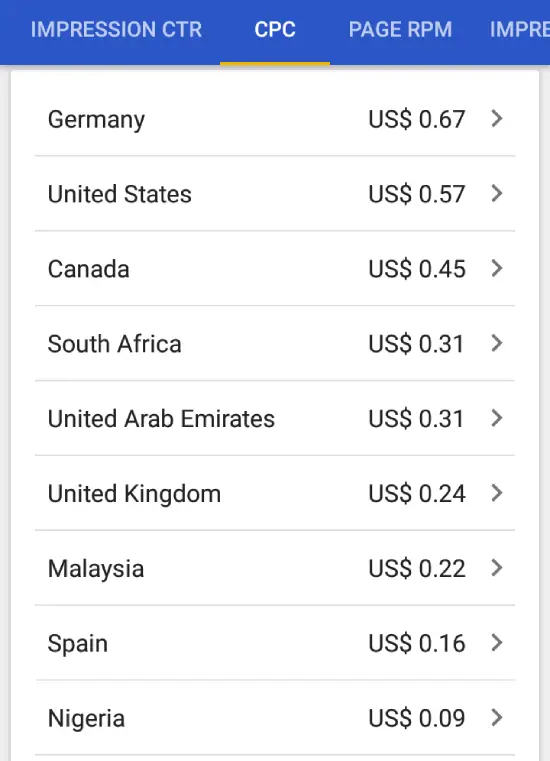The image shows a detailed screenshot of a pop-up box with a white background. This pop-up box is encased by a thin gray border on the left, right, and top sides. Above this gray border is a distinctive blue banner. The banner features prominently in white, uppercase text with various labels, including "IMPRESSION," "CTR," "CPC," "PAGE RPM," and "IMPR," though the latter is partially cut off at the right edge of the image.

Directly below the blue banner, a thin yellow horizontal line serves as a separation between the header and the main content of the pop-up box. The core section of the pop-up presents text in a column format with black font, enumerating several countries alongside specific monetary values. The list, segmented by thin gray horizontal lines, reads as follows:

- Germany: US $0.67
- United States: US $0.57
- Canada: US $0.45
- South Africa: US $0.31
- United Arab Emirates: US $0.31
- United Kingdom: US $0.24
- Malaysia: US $0.22
- Spain: US $0.16
- Nigeria: US $0.09